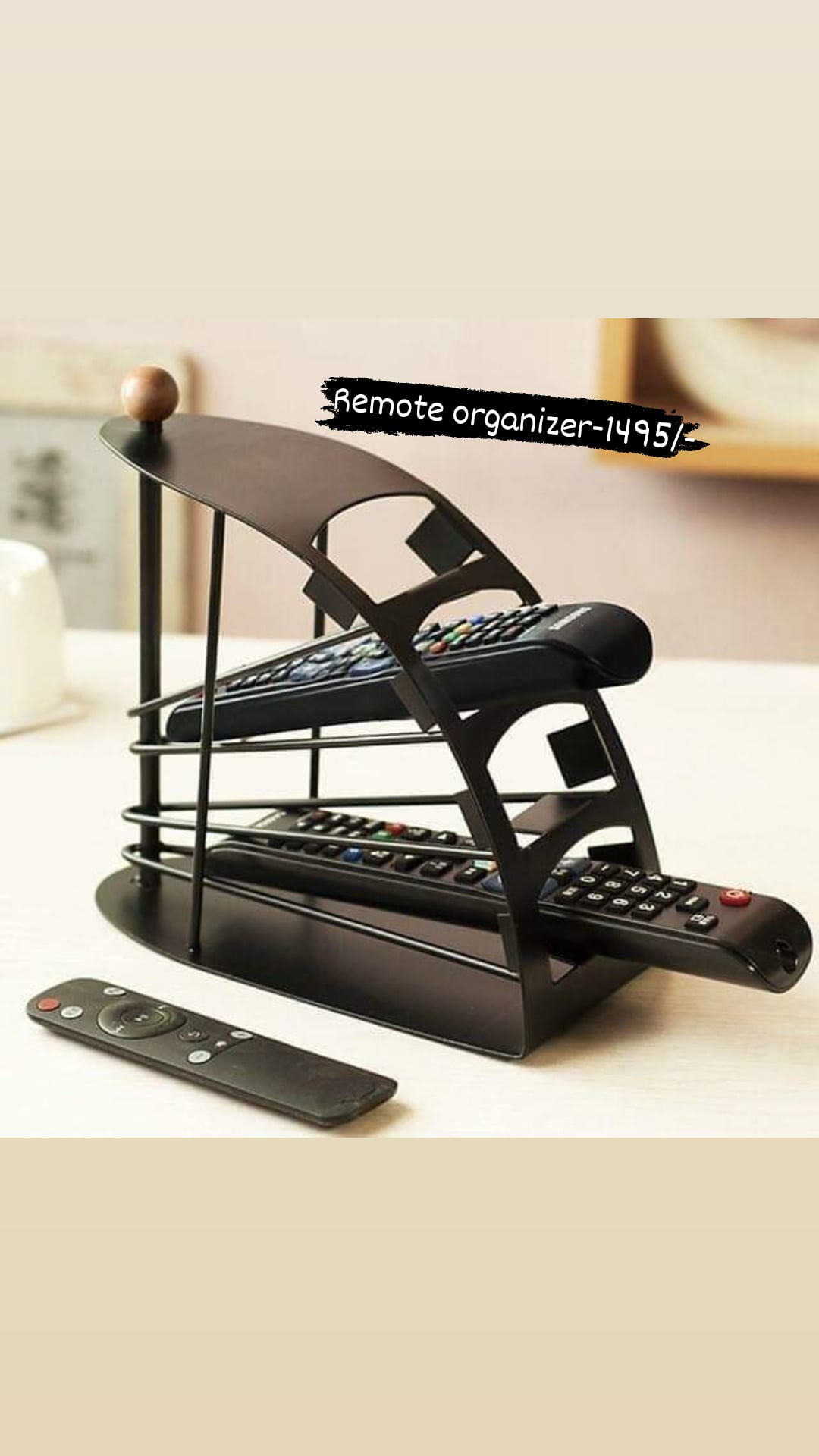The image depicts a custom-made remote control organizer, labeled "Remote Organizer 1495" in white letters against a black background. The organizer is constructed from black steel and wire with a base supporting a vertical structure that curves back at the top, resembling a car pedal. It has four slots designed to hold remote controls of various sizes. Two of the slots are occupied by long, button-covered remotes, one in the bottom slot and one in the third slot, while the second and fourth slots are empty. Additionally, a thin remote lies beside the organizer on a white office desk. The organizer's thin metal rods and stylish design ensure that the remotes rest securely, with each slot's angle gradually increasing upward. The photo is bordered by beige on the top and bottom, emphasizing the central focus on the well-crafted remote organizer.